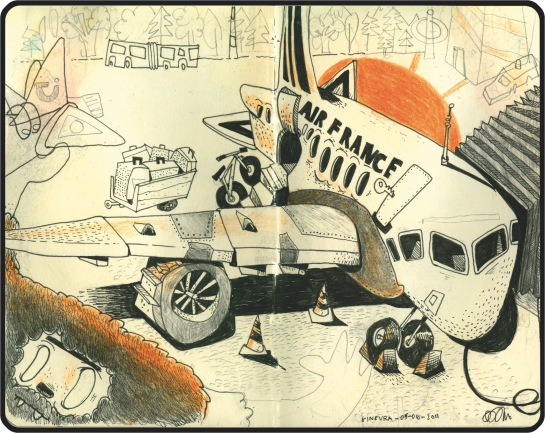The image is a detailed black, white, and orange comic book-style doodle featuring a large, distorted Air France passenger airplane facing the audience. The airplane's right wing is patched with steel plates along the base and middle, and there's a distorted jet engine beneath it. A luggage carrier full of suitcases is positioned next to the airplane, and the scene is bustling with airport activities, including two traffic cones, brakes around the front tire, and a vacuum or air ramp on the right-hand side. The background includes a bus and a line of trees, illuminated by an orange sun setting behind the airplane. In the bottom left-hand corner, there's a quirky, hairy character with big vacant eyes, a fur nose, two small fangs, a bushy beard/afro, and a unibrow, adding a playful element to the scene. The blend of cartoonish and detailed styles suggests it may be inspired by vintage Japanese sketches and possibly created by a French artist.